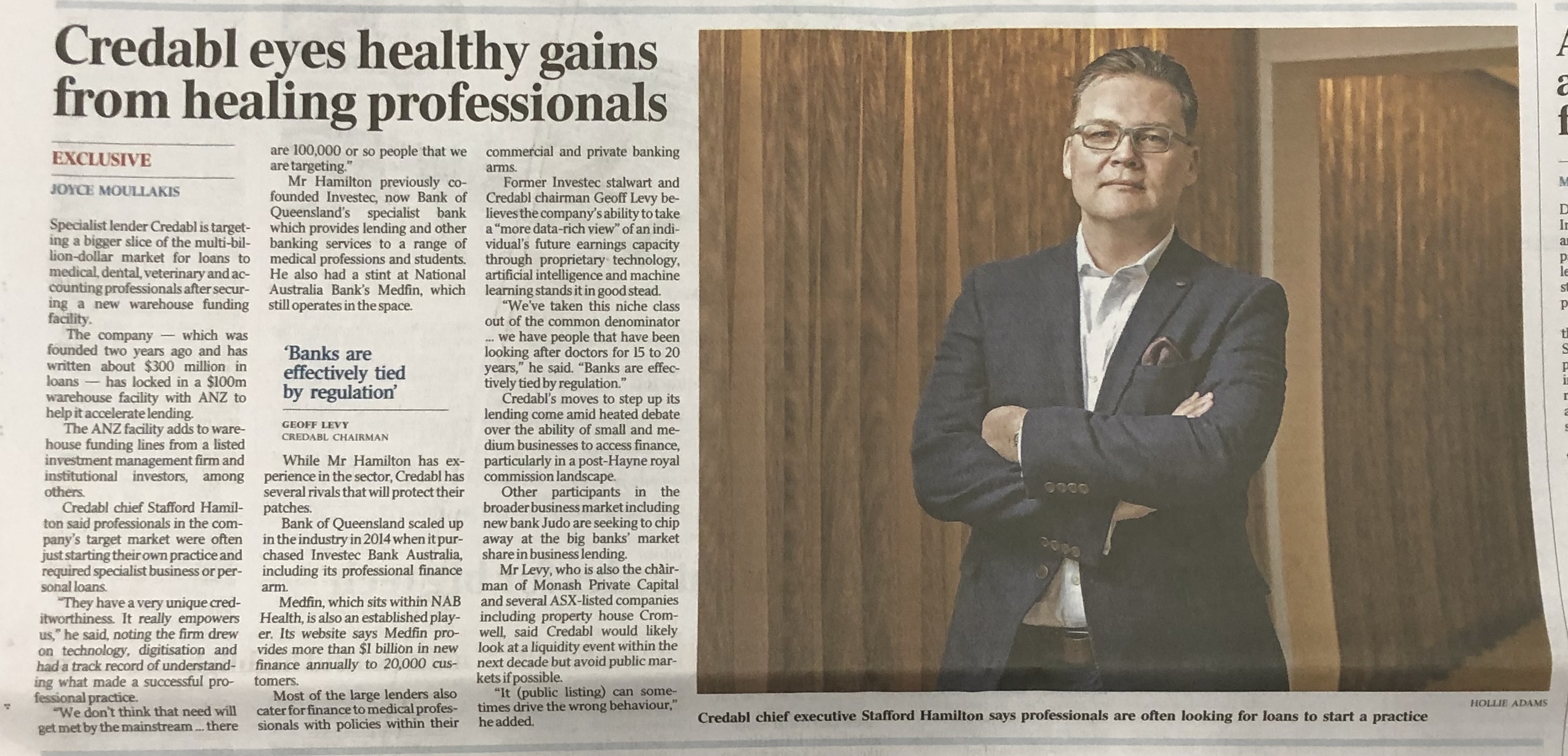The image features a cut-out newspaper article prominently displaying a photograph of a man. The man, a white individual, is dressed in a button-down shirt paired with a suit jacket adorned with a handkerchief in the pocket. He is wearing glasses, and his arms are folded confidently in front of him. A belt is discernible at his waist. The backdrop reveals a doorway and brown curtains over his right shoulder, indicating he is standing in an indoor setting.

The headline of the article prominently reads, "Credible Eyes, Healthy Gains from Healing Professionals," and is marked as exclusive. The author of the piece is noted, although the print is too small to be legible without close examination. Key phrases in the body of the article, such as "Banks are effectively tied by regulation," suggest a discussion about financial or regulatory viewpoints possibly tied to the subject's expertise.

The cut-out nature of the article is evident; the right-hand edge shows remnants of a neighboring article, the top and bottom edges are uneven, and the overall dimensions hint at hastiness in its removal, likely using scissors.